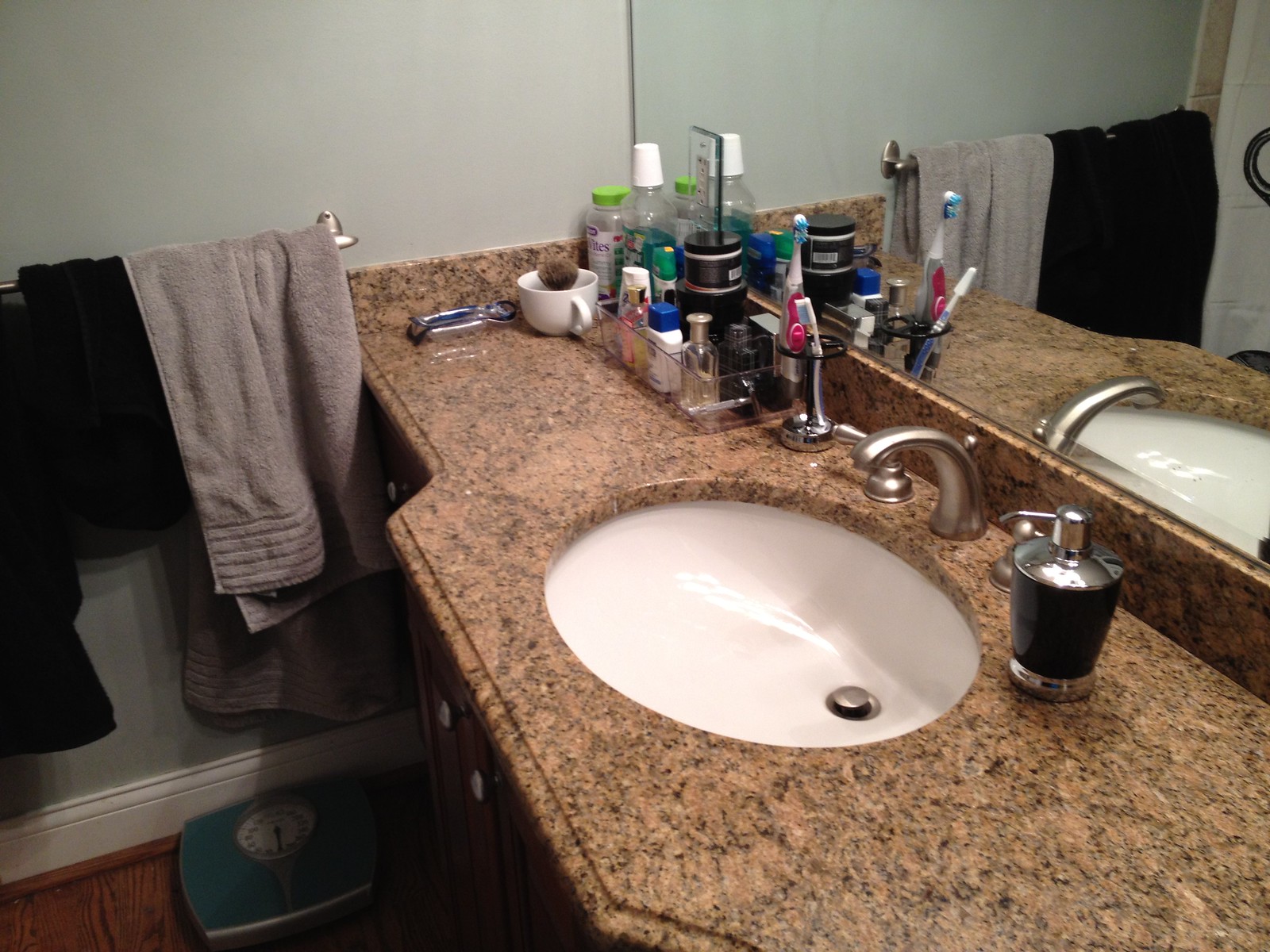This photograph captures a well-organized bathroom sink and its surrounding countertop in great detail. The main focus is the standard-looking sink, which features silver knobs on the left and a U-shaped silver spout positioned over the basin. The sink basin itself is white and includes a visible silver drainage pipe.

To the right of the handles for controlling the water flow sits a green soap dispenser. On the left side of the sink, a red and purple toothbrush is placed alongside various bottles, including one with a blue top and white bottom, a clear yellow bottle, and an orange-hued bottle, likely containing lotions or creams.

A mirror directly above the sink reflects the bathroom space, adding depth to the scene. To the far left of the image, two towels—a gray one and a black one—hang neatly, suggesting that more than one person uses the bathroom. Additionally, a non-electronic scale with a light blue top is visible in the bottom left corner, hinting at the personal care routines of the residents.

The overall setting is clean and functional, portraying a typical bathroom countertop arrangement.